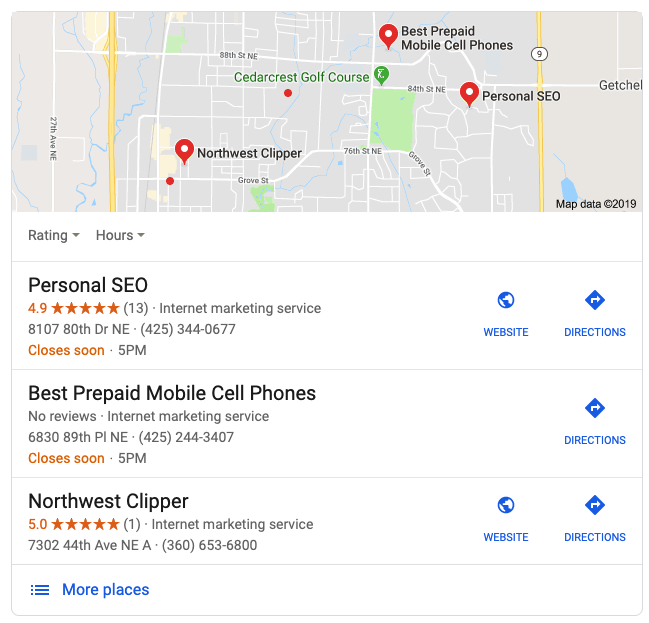The screenshot appears to be from Apple's Maps app, displaying a rectangular map that is wider than it is tall. The map showcases highways, streets, and labeled places, along with waterways marked in blue. 

Below the map, there are filters labeled "Rating" and "Hours," each accompanied by a down arrow for sorting or filtering options. 

The app also features three rows of listed locations: 
1. **Personal SEO**: Accompanied by buttons for "Website" and "Directions," each with respective logos.
2. **Best Prepaid Mobile Cell Phones**: Featuring a symbol followed by a "Directions" button.
3. **Northwest Clipper**: Includes buttons for "Website" and "Directions," each with logos and descriptive text beneath them.

At the screen's bottom, a footer contains three horizontal lines, each starting with a dot on the left. To the right of these lines, the text "More places" appears in blue, with a blue logo to the left.